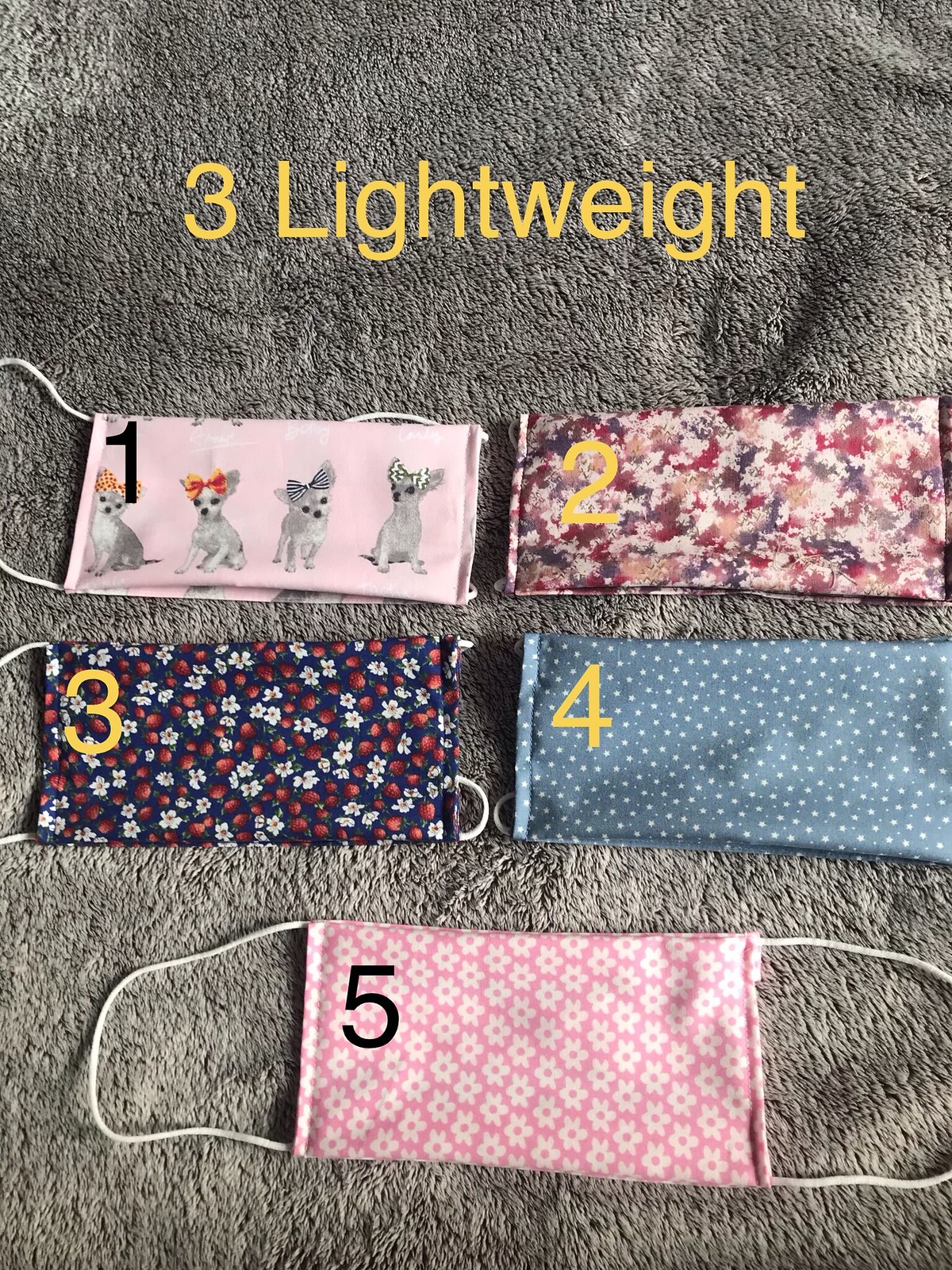This advertisement photo showcases a collection of five distinctive face masks, neatly laid out on what appears to be a large, fluffy gray towel. Each mask features a unique design, and they all have white elastic ear loops for wearing. 

Starting with the first mask, it stands out with its charming print of four chihuahuas adorned with bows, set against a pink background. The second mask displays an abstract, tie-dye pattern reminiscent of Jackson Pollock's artwork, blending shades of pink, gray, and white. The third mask features a delicate floral design with white flowers and red petals on a robust orange jacquard fabric, giving it a silky appearance. The fourth mask has a serene, desaturated blue background scattered with small white stars. The fifth mask pairs a pink backdrop with elegant white paisley flowers. 

At the top of the image, bold yellow numbers label each mask from one to five, and green text proclaims "3 Lightweight," highlighting the masks' comfortable, lightweight design, despite the fabric's sophisticated appearance.